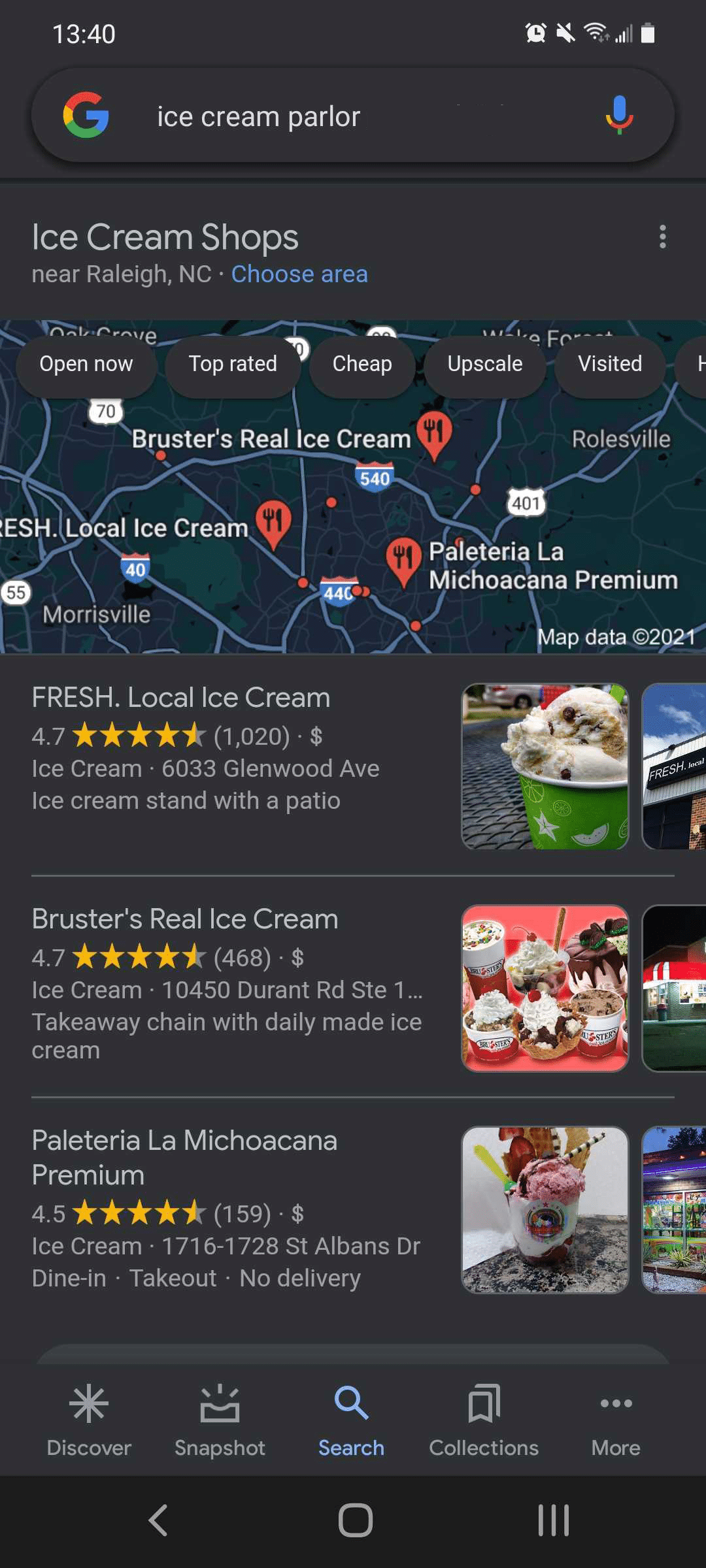The image depicts a Google search results page for "Ice Cream Parlor." At the top, the familiar Google logo is displayed, with the search query "Ice Cream Parlor" entered in the search bar. Beneath the search bar, the query refines to "Ice Cream Shops near Raleigh, North Carolina."

A map dominates the next section, marked with several red pins representing different ice cream shops. Each pin features an icon of a fork and knife. Notable locations pinpointed on the map include Bruster's Real Ice Cream, Local Ice Cream, and Palateria La Michoacana Premium. The map, which also shows various unnamed roads crisscrossing the area, is topped with tabs labeled "Open Now," "Top Rated," "Cheap," "Upscale," and "Visited," providing users with different filtering options.

Below the map, the first search result highlights "Fresh Local Ice Cream" located at 6033 Glenwood Avenue. It describes it as an "Ice Cream Stand with a Patio" and includes a photograph of a cup of ice cream.

The second result showcases "Bruster's Real Ice Cream," complete with its star rating and address. It is described as a "Takeaway Chain with Daily Made Ice Cream." The accompanying photo offers a visual of various ice cream products, including sundaes.

The third search result is "Palateria La Michoacana Premium," also featuring a star rating and address. It notes the options "Dine In," "Take Out," and "No Delivery." Beside this listing, there is a photo of some strawberry ice cream.